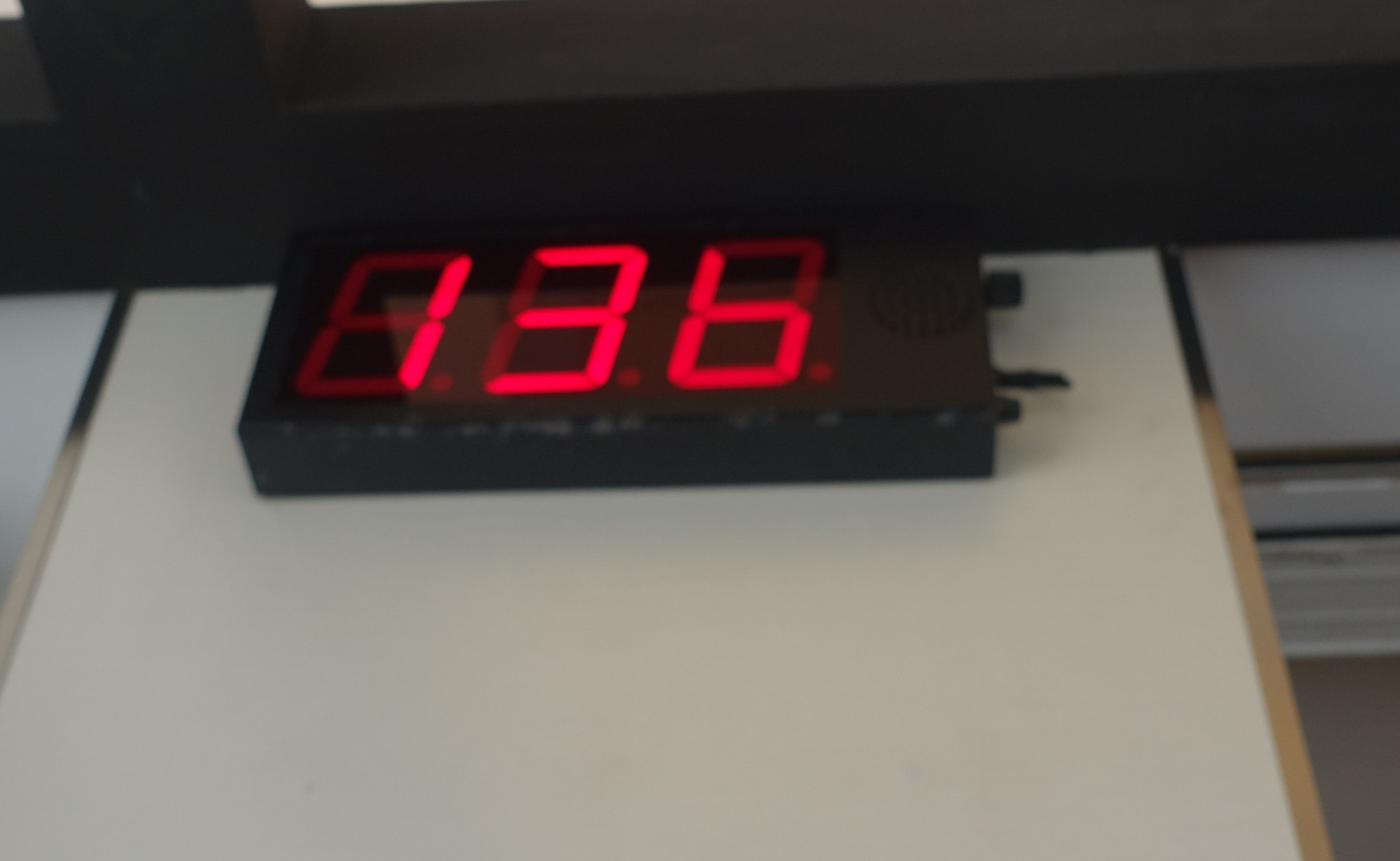The image depicts a large, beige wall with gold trimmings, and what appears to be a brown wooden panel accented with gold at the top. Beneath this wooden panel, a black digital clock is prominently displayed. The clock, which has a rectangular shape, shows red LED numbers reading "1:36." On the right side of the clock, there are two small black knobs and a circular speaker grid with holes. The lower right corner has another knob. The overall look hints at a timer clock, often used for timing activities. The white background wall behind this setup suggests it may be part of a more extensive installation, possibly close to the ceiling where some black elements can also be seen.